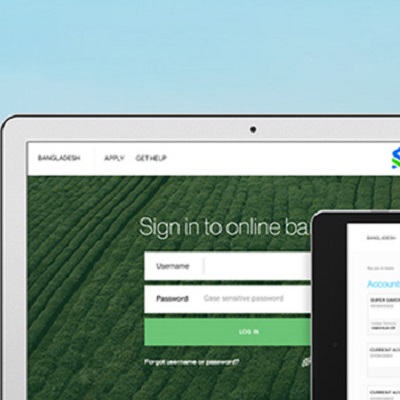This detailed caption describes the image as a magnified screenshot of a smartphone screen. The screenshot primarily focuses on the sign-in page for an online BA platform. At the top of the page, there are three tabs labeled "Bangladesh," "Apply," and "Get Help." Below these tabs, the page contains typical sign-in fields: a box for the username followed by a box for the password, which is noted to be case-sensitive. Beneath these fields is a green "Login" button.

The overall layout is juxtaposed against an aerial view of a lush green garden, which serves as the background. To the right side of the screen within the image, there is a small portion of a computer monitor visible, indicating that the screenshot was possibly taken on a laptop, and the smartphone image was then further zoomed in for clarity. The focus on the smartphone screen causes most other elements, including some text, to be nearly unreadable, contributing to the emphasis on the main sign-in content.